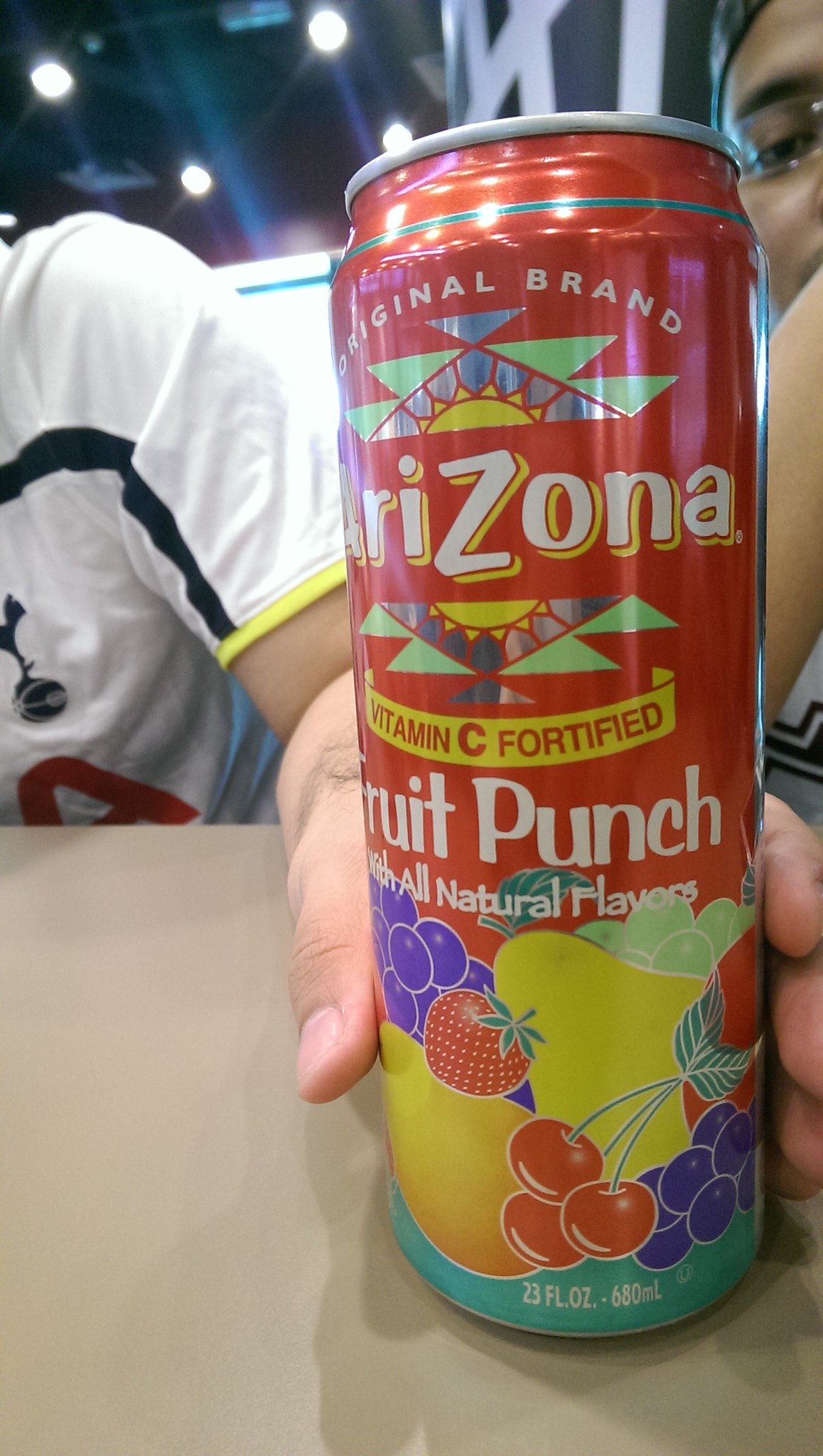In this close-up image, a hand lightly holds a vibrant red can of Arizona Fruit Punch, adorned with intricate designs and text. The can, prominently featuring a sun logo with yellow shapes, blue diamonds for the sky, and green triangles around it, boldly states "Original Brand" in white text at the top. Below the sun logo, the word "Arizona" is displayed in white text with a yellow shadow, though the 'A' is partially obscured by the curve of the can. Just beneath this, the sun symbol is repeated, followed by a yellow banner with red text declaring "Vitamin C Fortified." Further down, in white text, "Fruit Punch All Natural Flavors" stands out against a background transitioning from red to a vivid display of fruits, including grapes, lemons, pears, cherries, and strawberries. The bottom of the can features a light turquoise section with white text reading "23 FL OZ - 680 mL." 

The can rests on a light brown tabletop, with the tips of someone's fingers and thumb visible as they hold it. The person's shoulder, arm, and a bit of their torso can be seen in the background, along with another individual peeking into the frame, revealing parts of their face and arm. Both individuals appear to be indoors, as indicated by visible ceiling lights. The scene is detailed with the apparent attire: the person holding the can wears a white t-shirt with yellow edging on the sleeves, while the second person also wears a white shirt, though their design is less clear. The intricate detailing and branding make it a striking and informative visual of the Arizona Fruit Punch can amidst a casual indoor setting.